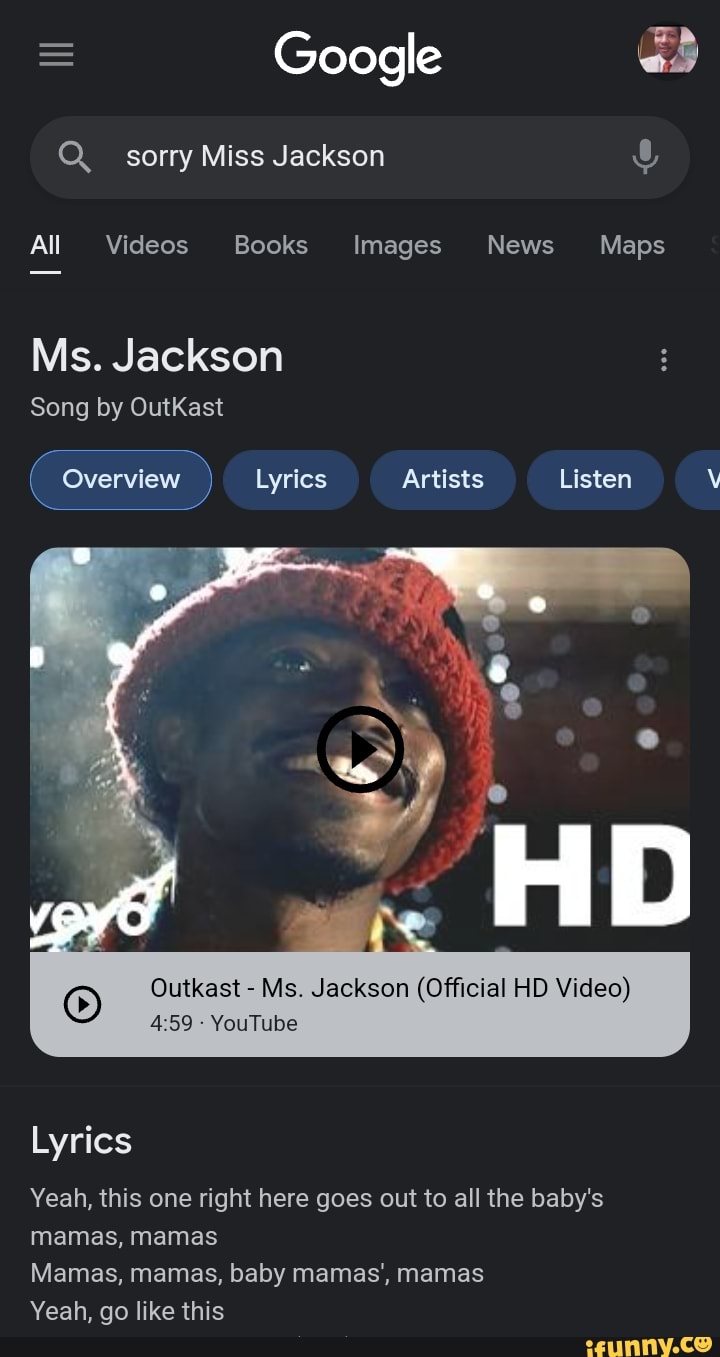This screenshot showcases a Google search performed in night mode, which features a dark grey background. The search query entered is "sorry Ms. Jackson," and the search categories available include All, Videos, Books, Images, News, and Maps. The top search result is a music-related entry for the song "Ms. Jackson" by Outkast.

The search result displays several interactive blue buttons labeled Overview, Lyrics, Artist, Listen, and a button with a "V," potentially for "View." Below these buttons, there is an embedded video player. The embedded video features a thumbnail image of one of the Outkast members smiling, with "HD" written in the font beside his face. He is wearing a red and black beanie and has a mustache and goatee. There is a black play button placed centrally on the image, which partially covers the artist's face.

The text below the video thumbnail reads "Outkast - Ms. Jackson (Official HD Video)," indicating the official music video from Outkast. The video is listed as being 4 minutes and 59 seconds long, hosted on YouTube, with a small play button icon on the left side.

Additionally, the result includes a brief snippet of the lyrics: "Yeah, this one's right here, goes out to all the babies, mamas, mamas, mamas, mamas, babies, mamas, mamas." Finally, at the bottom-right corner of the screenshot, there is a watermark or stamp from ifunny.co, identified by the icon "funny.ifunny.co" overlaid on the image.